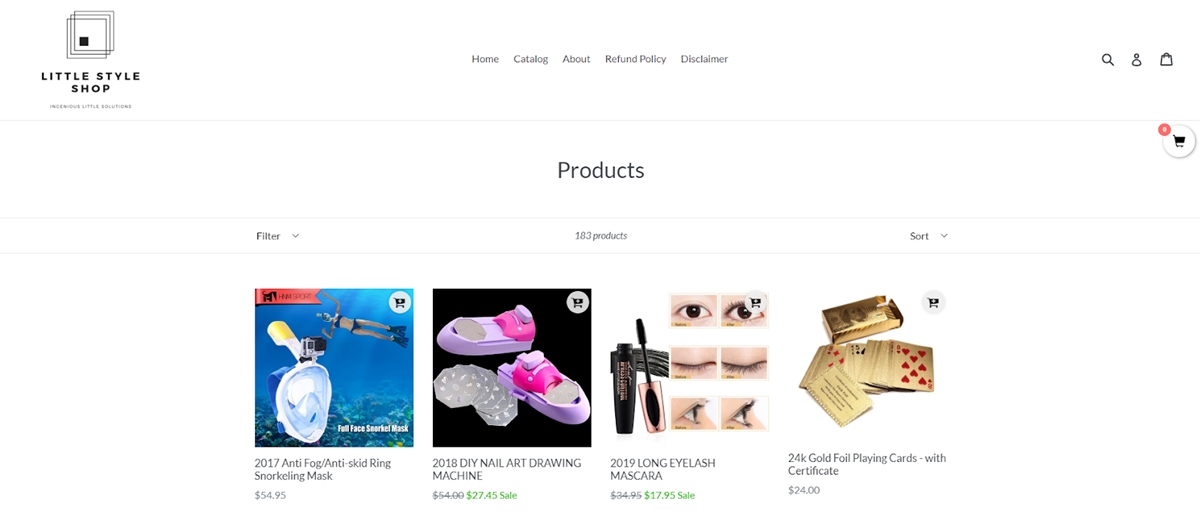The image depicts a webpage from the "Little Style Shop," identifiable by its logo located in the upper left-hand corner. The webpage features a white background with black text at the top, presenting a series of clickable tabs: Home, Catalog, Refund Policy, and Disclaimer. Below these tabs, there is a display of four products, each accompanied by distinctive descriptions and prices. The first product is labeled "2017 Anti-Fog Anti-Skid Ring Snorkeling Mask," priced at $54.95. The second item is an "2018 Do-It-Yourself Nail Art Drawing Machine," originally priced at $64.00 but currently on sale for $27.45. Following this is the third product, "2019 Long Eyelash Mascara," which has a regular price of $34.95 but is now available for $17.95. The final item in the lineup is a set of "24 Karat Gold Foil Playing Cards with Certificate," offered at $24.00.